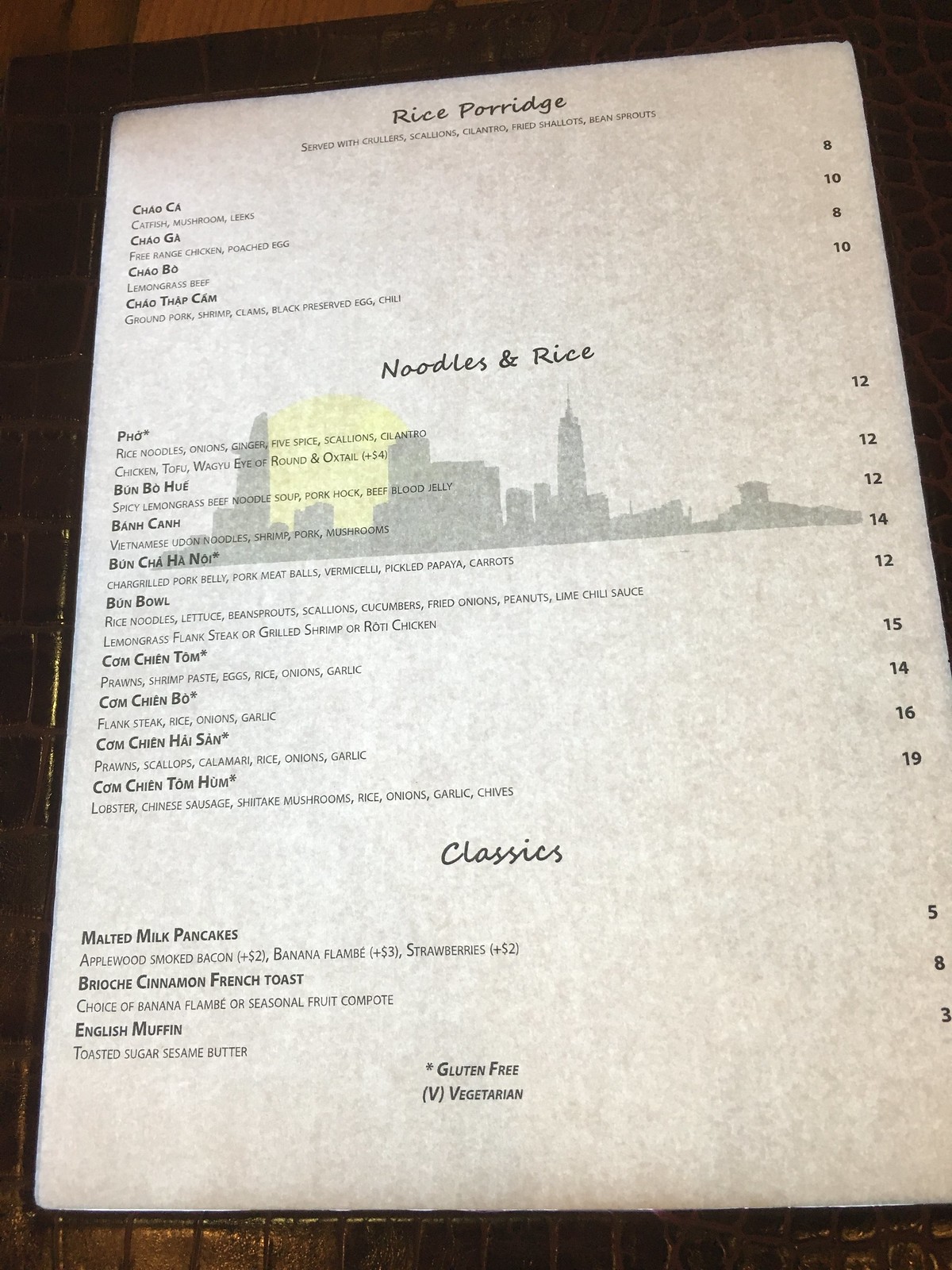The menu for this restaurant is intricately designed and printed on paper that has a textured, slightly weathered feel. At the top, the heading "Rice Porridge" is prominently displayed, introducing the first section of the menu.

**Rice Porridge:**
1. *Chow Ha:* Catfish, mushroom, and leeks.
2. *Chow Ga:* Free-range chicken with a poached egg.
3. *Chow Bo:* Lemongrass beef.
4. *Chow Thot Com:* Ground pork, shrimp, clams, black preserved egg, and chili.

**Noodles and Rice:**
1. *Pho:* Rice noodles with onions, ginger, five spice, garlic, cilantro, chicken, tofu, wagyu beef, and an optional oxtail addition for $4.
2. *Bun Bo Hue:* Spicy lemongrass beef noodle soup with pork hock and beef blood jelly.
3. *Banh Canh:* Vietnamese udon noodles with shrimp, pork, and mushrooms.
4. *Bun Cha Hanoi:* Chargrilled pork belly, pork meatballs, minced pork, pickled papaya, carrots.
5. *Bun Bo:* Rice noodles with lettuce, bean sprouts, scallions, cucumbers, fried onions, peanuts, lime, chili sauce, and your choice of lemongrass flank steak, grilled shrimp, or roti chicken.
6. *Com Tom:* Prawns with shrimp paste, eggs, rice, onions, and garlic.
7. *Com Bo:* Flank steak with rice, onions, and garlic.
8. *Com Hai San:* Prawn, scallops, and calamari with rice, onions, and garlic.
9. *Com Tom Hun:* Lobster with Chinese sausage, shiitake mushrooms, rice, and Scotch fries.

**Classics and Extras:**
1. Multiple varieties of pancakes. (Smoked bacon is an additional $2)
2. Banana flambé ($3), strawberries ($2), or seasonal fruit compote.
3. Brioche cinnamon French toast.
4. English muffins with toasted sugar sesame butter.

Throughout the sections, the background of the menu features a grayscale print of the city's skyline with the sun setting behind it, creating silhouettes of buildings. Notes indicate gluten-free and vegetarian options are available.